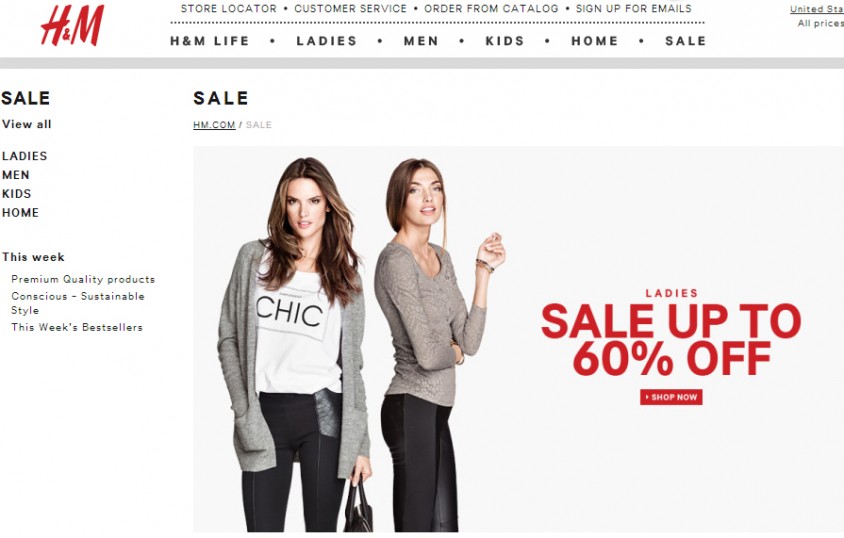This image captures a snapshot of the H&M website, which specializes in fashion and clothing. Dominating the center of the webpage are two strikingly attractive young women, both brunettes with long hair, showcasing stylish outfits. They are wearing fitted black pants paired with gray, long-sleeved sweaters. To the right of this image, bold red text announces, "Ladies, sale up to 60% off, shop now," enticing visitors to explore the sale.

On the left side of the webpage is a sidebar menu presenting various categories of sale items, with options to view all or to filter by ladies, men, kids, and home. Across the top, the navigation bar includes tabs such as "Store Locator," "Customer Service," "Order from Catalog," and "Sign Up for Emails," providing users with easy access to essential services. Just below this navigation bar, additional options like "H&M Life," "Ladies," "Men," "Kids," "Home," and "Sale" are available for browsing.

In the upper right-hand corner of the page is a small informational block clarifying that all displayed prices are in U.S. dollars, catering to users in the United States.